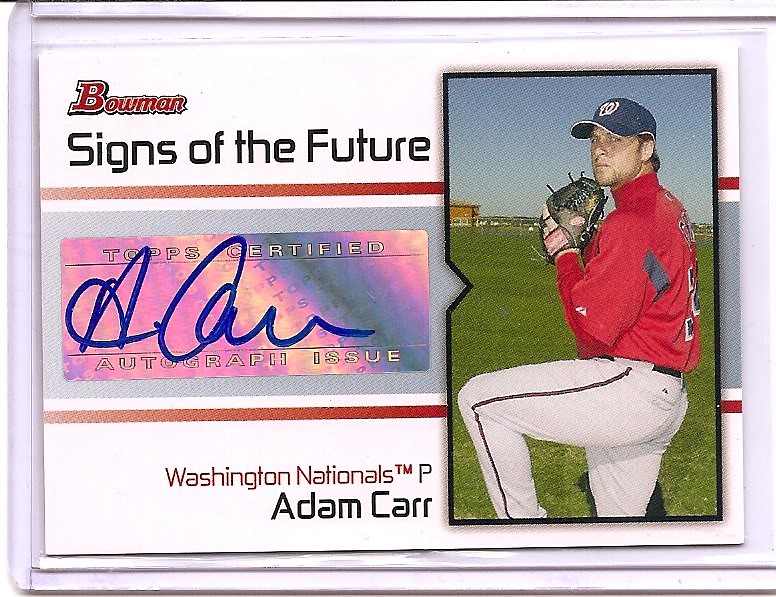This image features an autographed, collectible baseball card issued by Bowman, titled "Signs of the Future." The card highlights Adam Carr of the Washington Nationals. In red lettering, "Bowman" appears in the upper left corner, followed by "Signs of the Future" below it. The top center region of the card showcases the certification from Topps, reading "Topps Certified" and "Autograph Issue," with Adam Carr's blue-ink signature. The player's name, "Adam Carr," along with "Washington Nationals" and a "P" for pitcher, are printed on a white band at the bottom. The card is structured in three horizontal sections, with the right half displaying a photograph of Adam Carr in his Washington Nationals uniform—a dark navy blue cap with a cursive W, a red short-sleeved game shirt with a red turtleneck, white pants with a dark stripe, and a black glove. Carr appears poised to pitch, with his left knee lifted and his hand near his chin, emanating a serious and focused demeanor. The card is bordered and sectioned by pink and red layers, with additional red lines dividing the horizontal segments. The overall design is marked by swirly, rainbow-like colors, adding a holographic effect.